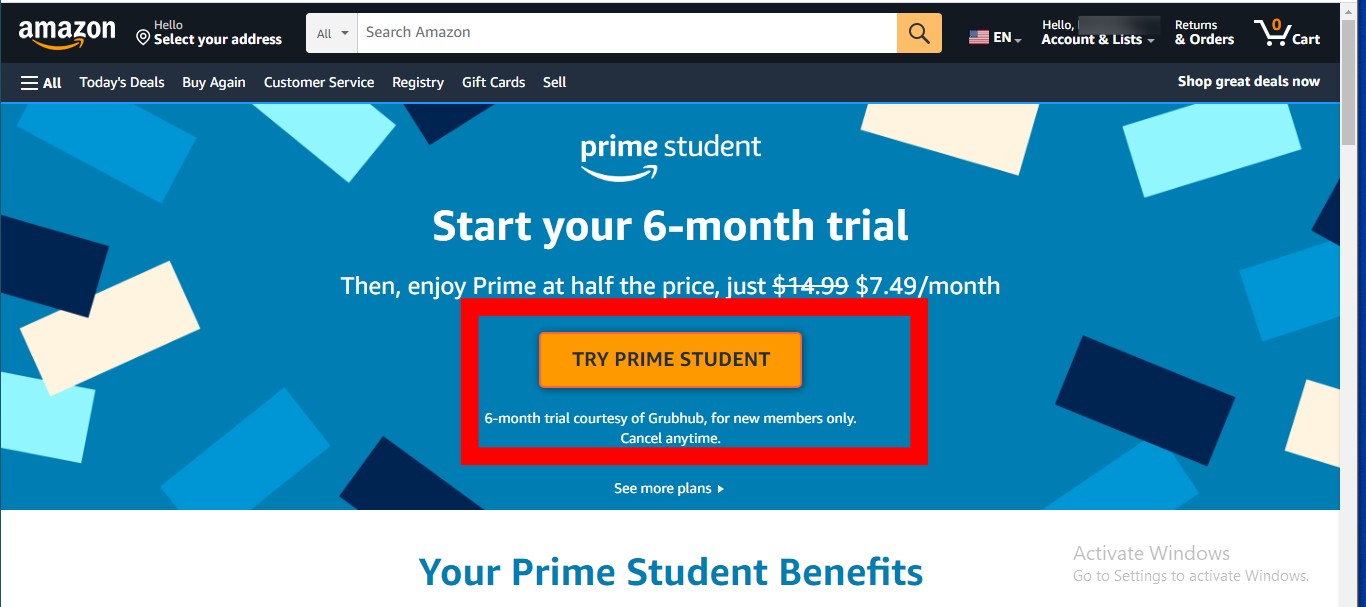The screenshot captures the Amazon Prime Student section of the Amazon website, structured methodically with detailed headers and promotional content.

**Header Section:**
- Across the top, there's a dark bar with standard Amazon elements. The leftmost side features the Amazon logo in white, accompanied by the signature yellow arrow beneath it. Adjacent to the logo, the text "Hello, select your address" is displayed.
- Next is a search field, which includes a category filter drop-down menu on the left, a central input area labeled "Search Amazon," and a right-aligned yellow search button with a dark magnifying glass icon.
- To the right of the search bar, the language selection is set to English (EN), indicated by the US flag.
- Following this are the user account options, starting with a blurred-out user name, followed by "Account & Lists," "Returns & Orders," and a shopping cart icon with "0" items, denoted in yellow next to the word "Cart".

**Submenu Section:**
- Below the main header, a dark blue sub-menu strip features various navigation options in white text: a three-line hamburger menu icon, "All," "Today's Deals," "Buy Again," "Customer Service," "Registry," "Gift Cards," "Sell," and an emphasized "Shop great deals now" on the far right side.

**Hero Section:**
- The main promotional area below the headers showcases an abstract, geometric design with blue and white shapes. Central to this backdrop is the Prime Student logo in white.
- The promotional text announces: 
  - "Start your 6-month trial" in large white letters,
  - Followed by "Then enjoy Prime at half price just $14.99" (struck through) with "$7.49 a month" beneath it.
- A prominent yellow button with slight shadowing reads "TRY PRIME STUDENT" in capital letters, highlighted by a thick red rectangle added by the user. 
- Below the button, small text clarifies: "Six-month trial courtesy of GrubHub for new members only. Cancel anytime."

**Content Section:**
- Beneath the promotional section, the background transitions to white. Centered text in blue reads "Your Prime Student Benefits."
- A watermark notification in the lower right corner notes: "Activate Windows, Go to Settings to activate Windows."

This styled webpage image effectively promotes the Prime Student membership, offering clear navigation and enticing trial benefits.